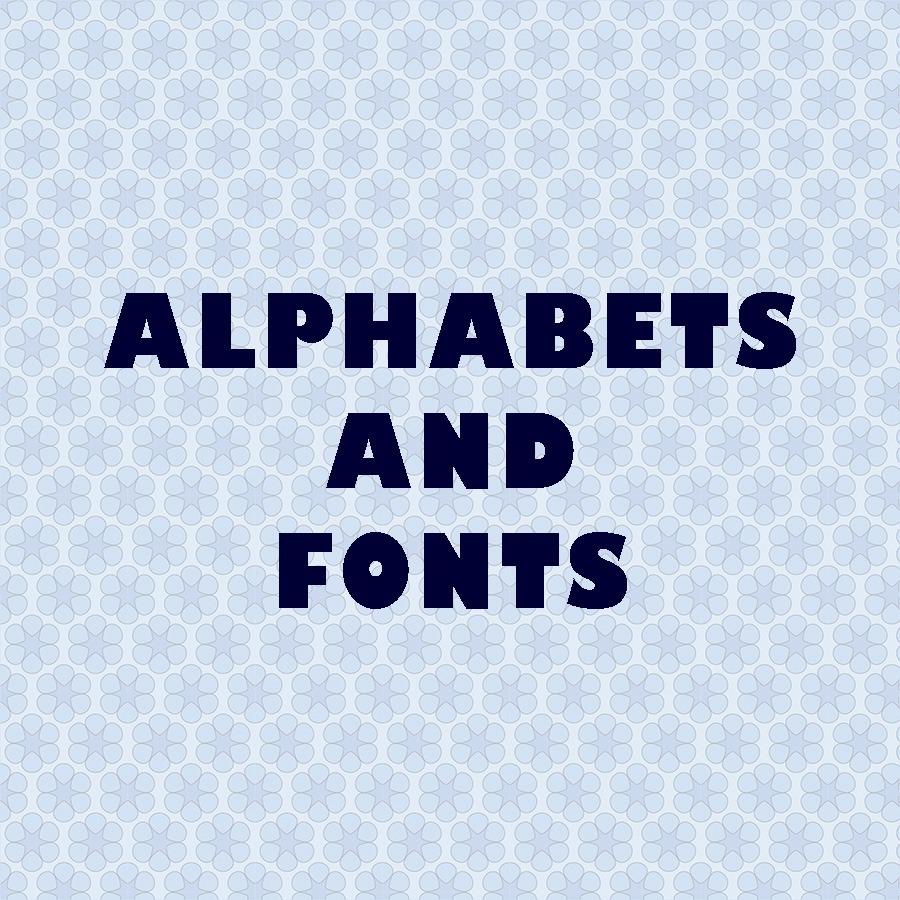The poster features a prominent title, "ALPHABETS AND FONTS," centered in all caps and bold dark blue font against a meticulously patterned light blue background. The background consists of a tiled design with approximately 252 flower-like shapes cascading across the entire canvas. Each flower, composed of six blue petals extending from the gaps of six-point stars, forms a complex and harmonious pattern. These flowers are organized in 18 columns ascending the left side and 14 rows extending to the right, with each subsequent row offset so the top petal of each flower aligns just below the gap of two flowers above. The minimalist yet intricate design of the poster combines both elegance and precision, creating a visually compelling piece.